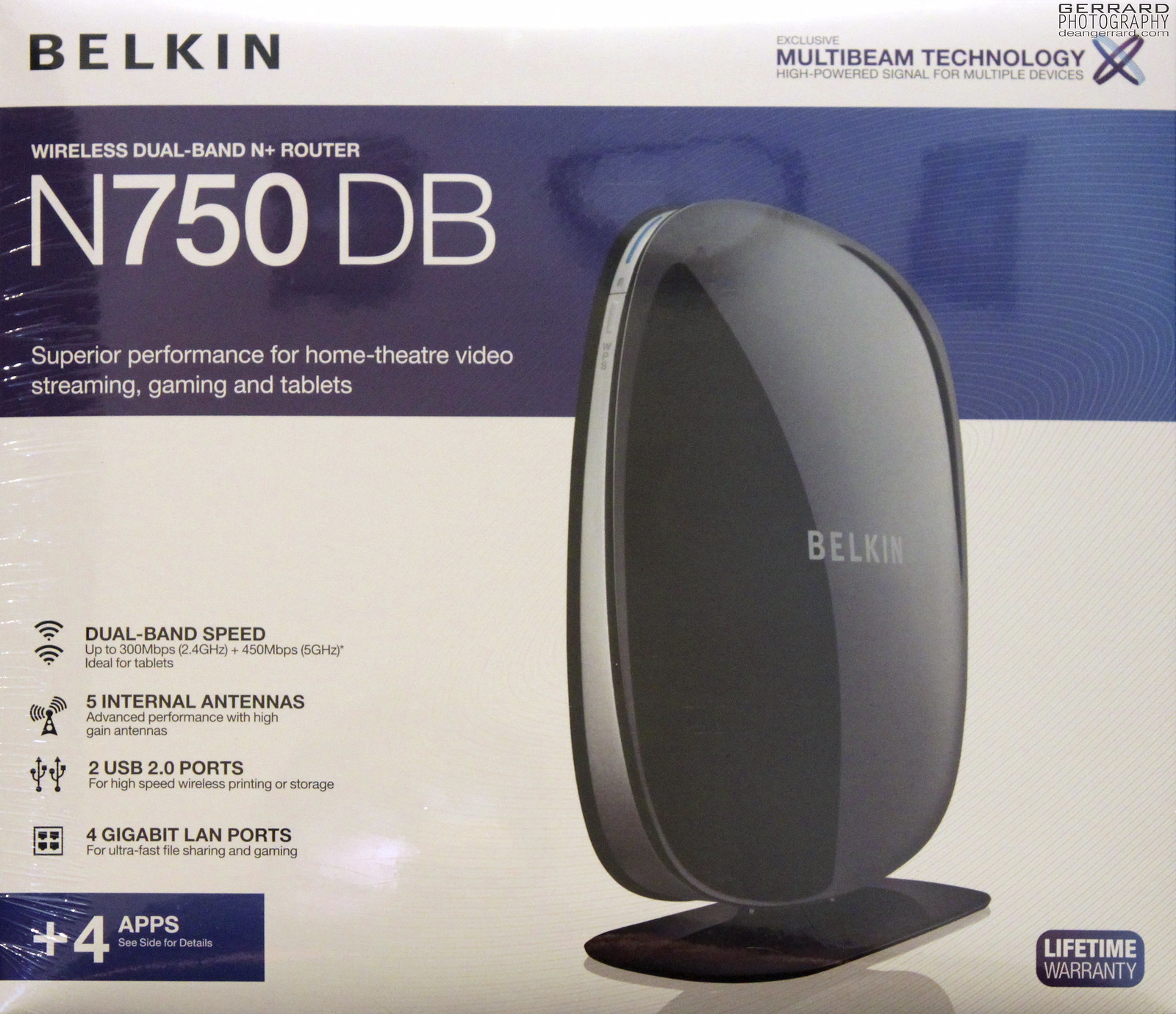The image displays the front of a packaging box for a Belkin wireless dual-band N+ router, specifically the N750DB model. Dominating the right half of the box is a large, shiny black router mounted on a stand. The upper left corner features a white rectangle with black text reading "Belkin." Adjacent to it, the upper right corner touts the router’s "exclusive multi-beam technology" and claims "high-powered signal for multiple devices." A watermark labeled "Girard Photography, deangirard.com" is also visible in the top right. Along a prominent blue border near the top, white text highlights the router's model and promises "superior performance for home theater, video streaming, gaming, and tablets." Additional details along the bottom right confirm a lifetime warranty, while the bottom left notes the inclusion of "plus four apps." Key specifications are listed prominently, including "dual-band speed, five internal antennas, two USB 2.0 ports, and four gigabit LAN ports," with respective icons for each feature enhancing the informative design.